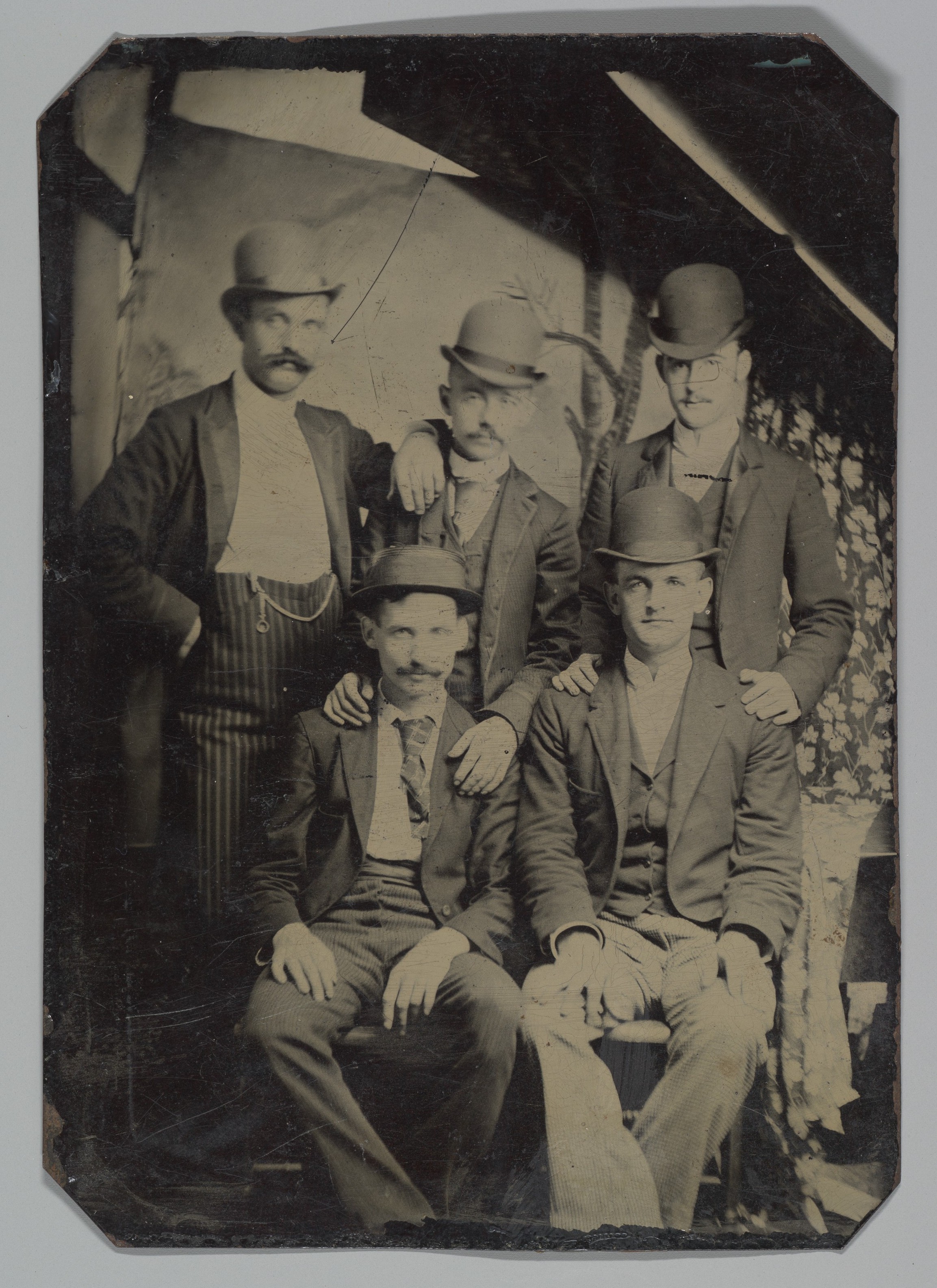This is a black and white antique photograph likely from the early 20th century, featuring five men posed together in a studio setting with a painted backdrop of trees and flowers. The two men sitting in front wear three-piece suits, with one sporting a pocket watch and striped patterned pants, while the other wears a tie. Behind them stand three men, all with mustaches and dressed in fine period attire, including suits and brimmed hats with ribbons. The men in the back have their hands resting on the shoulders of those in front, one with his arm laid over the man's shoulder beside him. All five men are smiling pleasantly, suggesting camaraderie. The backdrop, resembling a scene with flowers and trees, adds an artistic touch to the studio portrait. The entire photograph has an aged, yellowed appearance, indicative of its vintage origin.